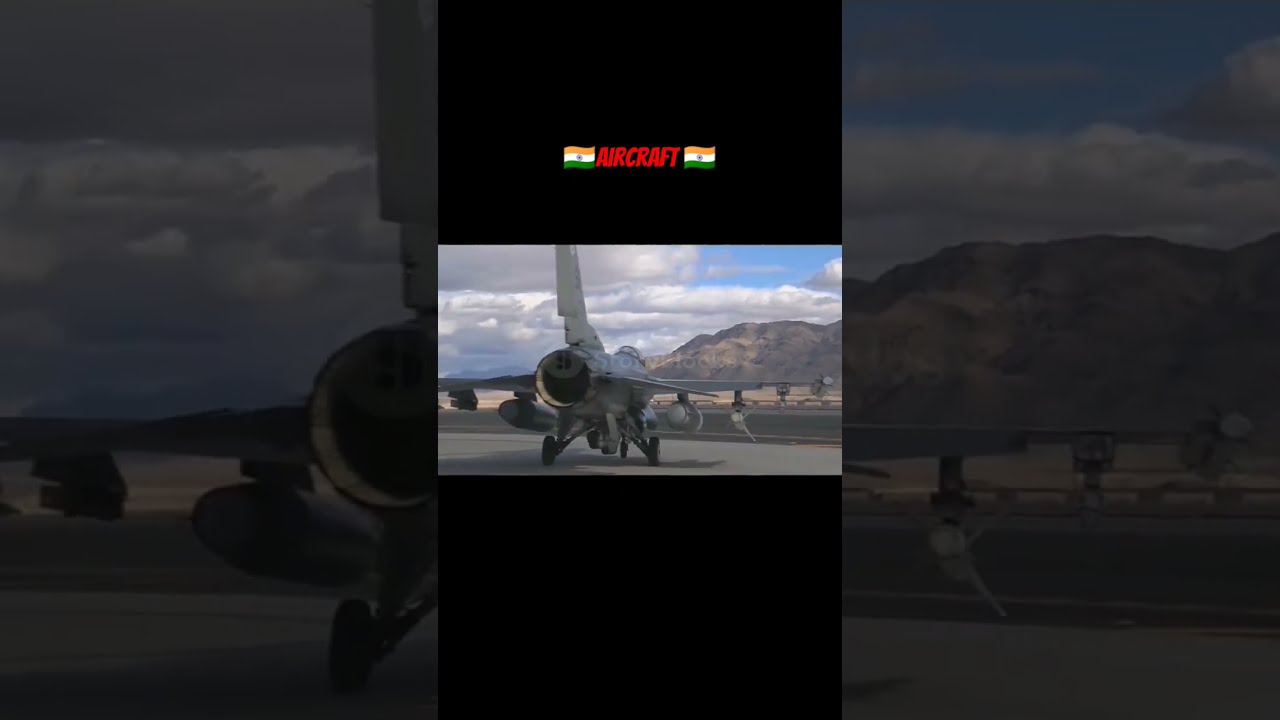The image is a slightly blurry, washed-out digital photograph of the back of a silver-gray fighter jet. The jet is parked on a tarmac, situated in a desert-like area with beige and purplish mountains framed by a soft light blue sky and layered white clouds in the background. The aircraft features a large singular exhaust port and visible weaponry, including two missiles—one large and singular, the other thin and elongated. There is an indistinct watermark across the image. Above the plane, there is bold, red, italicized text that reads "aircraft," flanked on either side by Indian flags, recognizable by their orange, white, and green stripes with a distinctive logo in the center of the white stripe. The ground where the jet is positioned has a greenish marble appearance.